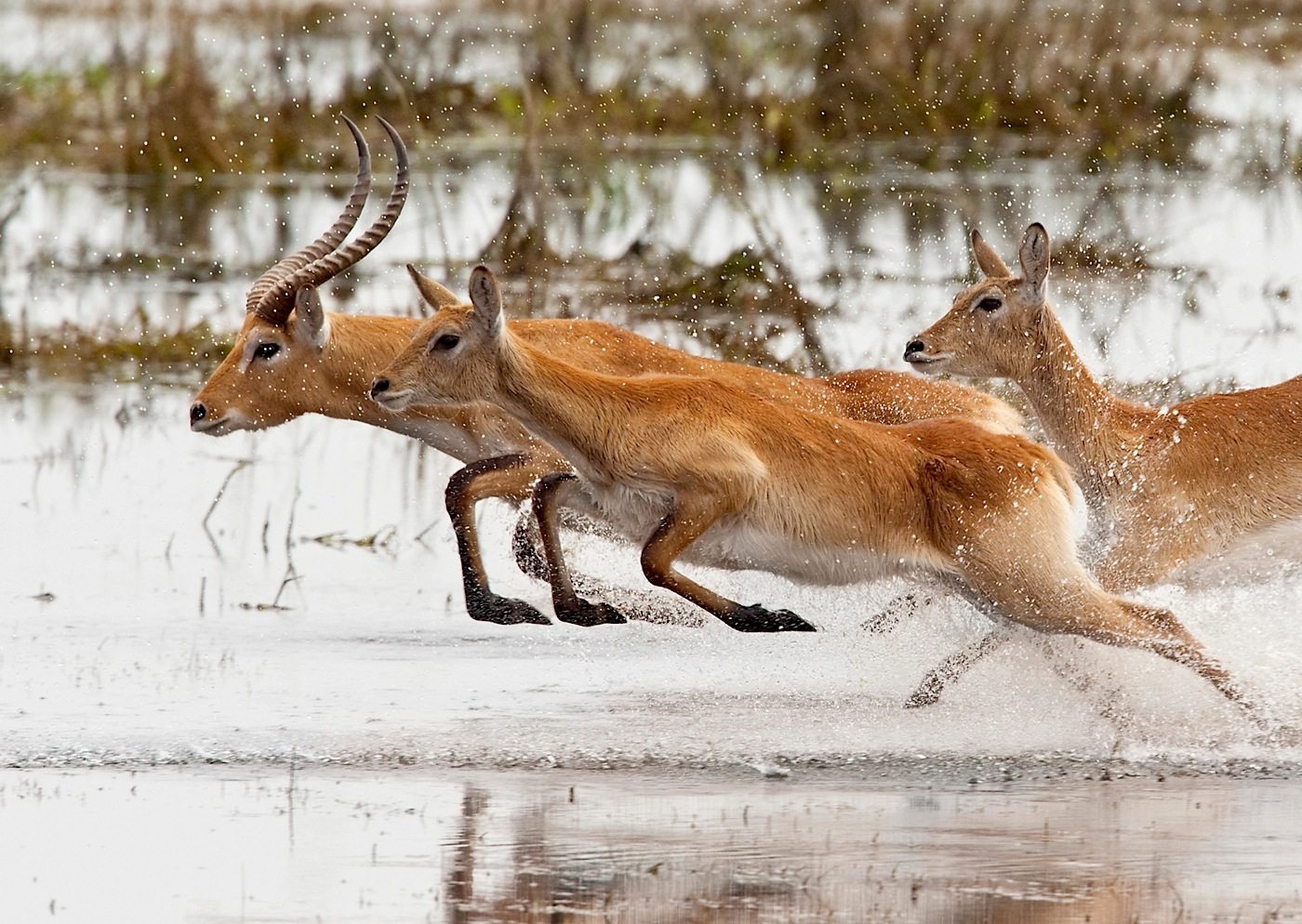A horizontal image captures three tan-colored deer running swiftly through a snow-covered landscape. The scene is bright, indicating daytime, and it appears to be either snowing or raining, giving the ground a wet and reflective appearance. One deer prominently features long, ribbon-like horns curving back and forward, while the other two, which are likely female or younger deer, lack antlers and display only ears. All three deer are airborne, their hooves kicking up shallow water as they move. In the blurred background, patches of water interspersed with greenish-brown plants can be faintly seen amidst the snowy terrain.